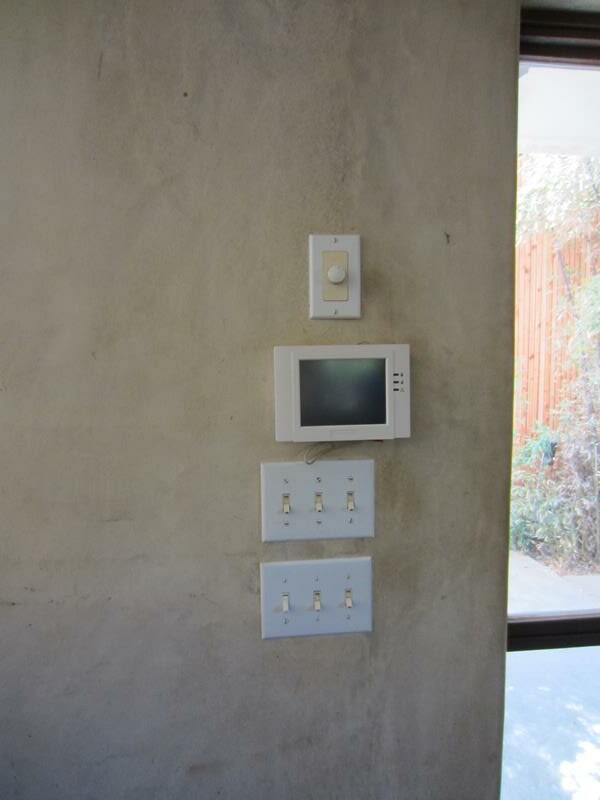The photograph showcases a textured, bumpy gray cement wall occupying the majority of the frame. On the right side, a large window spans the length of the wall. The window is divided into sections by black horizontal and vertical lines. Through the window, the outdoors is visible, featuring a grassy area, a brown fence adorned with flowers and leaves.

Starting from the top of the gray wall, there is a white electrical outlet with a rectangular base. Below it, there is an electronic thermostat with a white border and a gray screen. Further down, there are two identical white light switches, each with three switches neatly aligned.